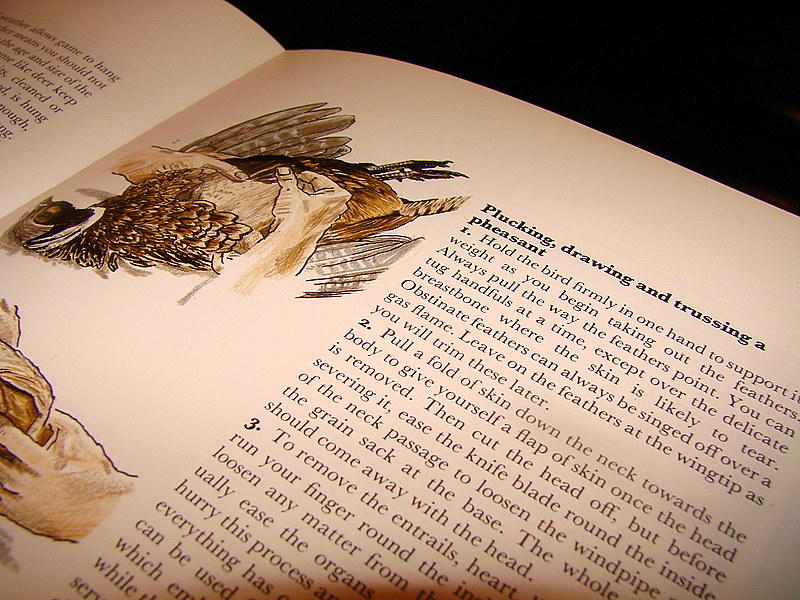This photograph captures a page from a classic cookbook that's dedicated to the process of plucking, drawing, and trussing a pheasant. The page is slightly turned to the right, presenting the text diagonally from the bottom left to the top right. The sepia-toned page features a title at the top in bold black letters, "Plucking, Drawing, and Trussing a Pheasant." The right column of the page contains detailed, numbered instructions on how to perform the tasks. The first paragraph advises holding the bird firmly and removing the feathers by pulling them in the direction they point. The second section describes pulling a fold of skin down the neck towards the body to create a flap once the head is removed. The third paragraph begins instructions on removing the entrails but is cut off in the photograph. The left column showcases intricate illustrations of hands holding a pheasant, depicting the plucking, drawing, and trussing process. These illustrations are drawn in brown and add an artistic touch to the instructional manual. The page exudes a vintage charm and provides a glimpse into traditional culinary techniques.